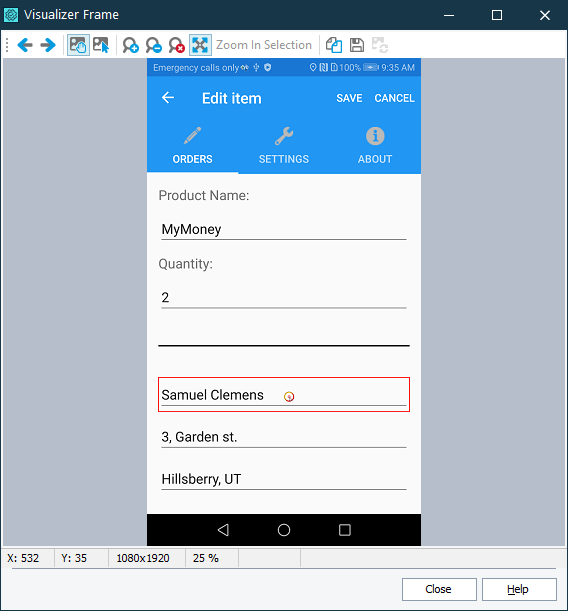This is a screen capture from an application named Visualizer Frame, which seems to be a Windows software or possibly a mobile app adapted for desktop use. Within this window, there is a smaller, phone-sized image displaying an interface for editing an item in an app other than Visualizer Frame. The smaller image's interface is titled "Edit Item." Below this title, the interface features options such as "Orders," "Settings," and "About." 

Further down, there is a text field labeled "Product Name" containing the text "My Money." Another text field labeled "Quantity" follows, with the text "To." Underneath these fields, there is a highlighted address, specifically the name "Samuel Clemens," enclosed in a red rectangle for emphasis. The address continues on the subsequent lines, stating "3 Garden Street" and "Hillsbury, UT."

Surrounding the embedded phone interface within the Visualizer Frame application, various control options are visible. These include navigation buttons for moving back and forth, zoom-in and zoom-out buttons, as well as a save button, a close button, and a help button.

This detailed setup offers a clear view of the nested interface within the Visualizer Frame application, showcasing its capabilities for editing and managing other applications or items.